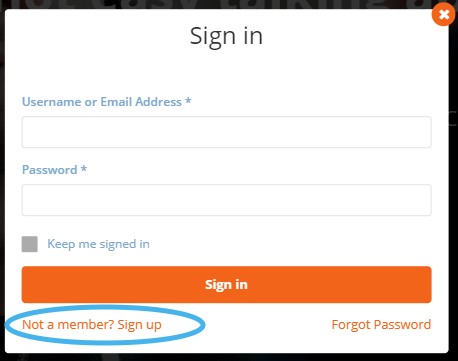A screenshot of a standard sign-in page is displayed, primarily characterized by its centered alignment and sleek, minimalistic design. The page features a clean, black margin that frames the interface. At the top right corner, an orange "X" button allows users to exit the page if they choose not to proceed.

Central to the page are two text fields, one for entering a username or email address and the other for a password. Below these fields is a checkbox option labeled "Keep me signed in," providing convenience for future logins. The primary call-to-action button, "Sign In," matches the orange color of the "X" button, ensuring visual consistency.

At the bottom of the page, an option is prominently circled: "Not a member? Sign up," which invites new users to create an account, though it comes with the typical annoyance of potentially frequent email notifications. To the right of this is a "Forgot Password?" link for users who may have an existing account but have trouble remembering their login details.

This type of mandatory sign-up/sign-in page can often be a barrier, preventing users from accessing content without committing to an account creation process.